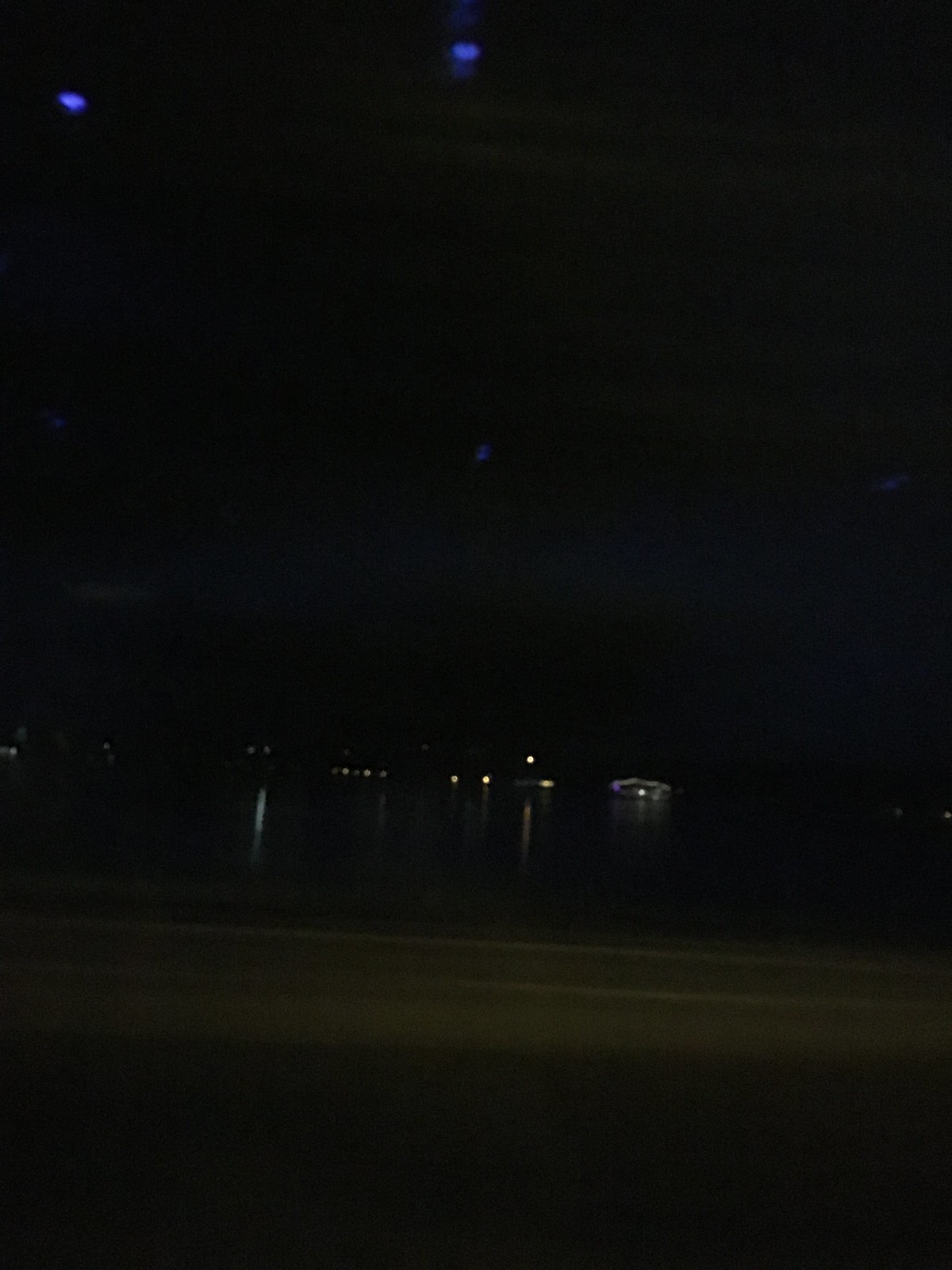The photograph depicts a very dark and blurry nighttime scene, capturing an outdoor setting where visibility is minimal due to the darkness. In the foreground, the image is dominated by shadowy, dark gray blurs and indistinct lines. A faint yellow blur with black lines appears to demarcate a boundary, possibly of a beach or shoreline. There are assorted dots and specks scattered throughout the image.

At the top portion of the picture, small, round blue lights form a pattern that could potentially be part of a distant light post arrangement, though the supports aren't visible. Further back, the scene is dotted with clusters of lights of varying colors—yellow and orange—likely indicating homes or small buildings spread out with gaps in between.

In addition to these, the sky above features scattered, small purple oval shapes floating amidst the pitch-black and gray, creating an almost eerie atmosphere. Reflective patterns on what is surmised to be water suggest the presence of boats or structures casting their glimmers onto the surface, enhancing the sense of tranquil yet mysterious nighttime environment.